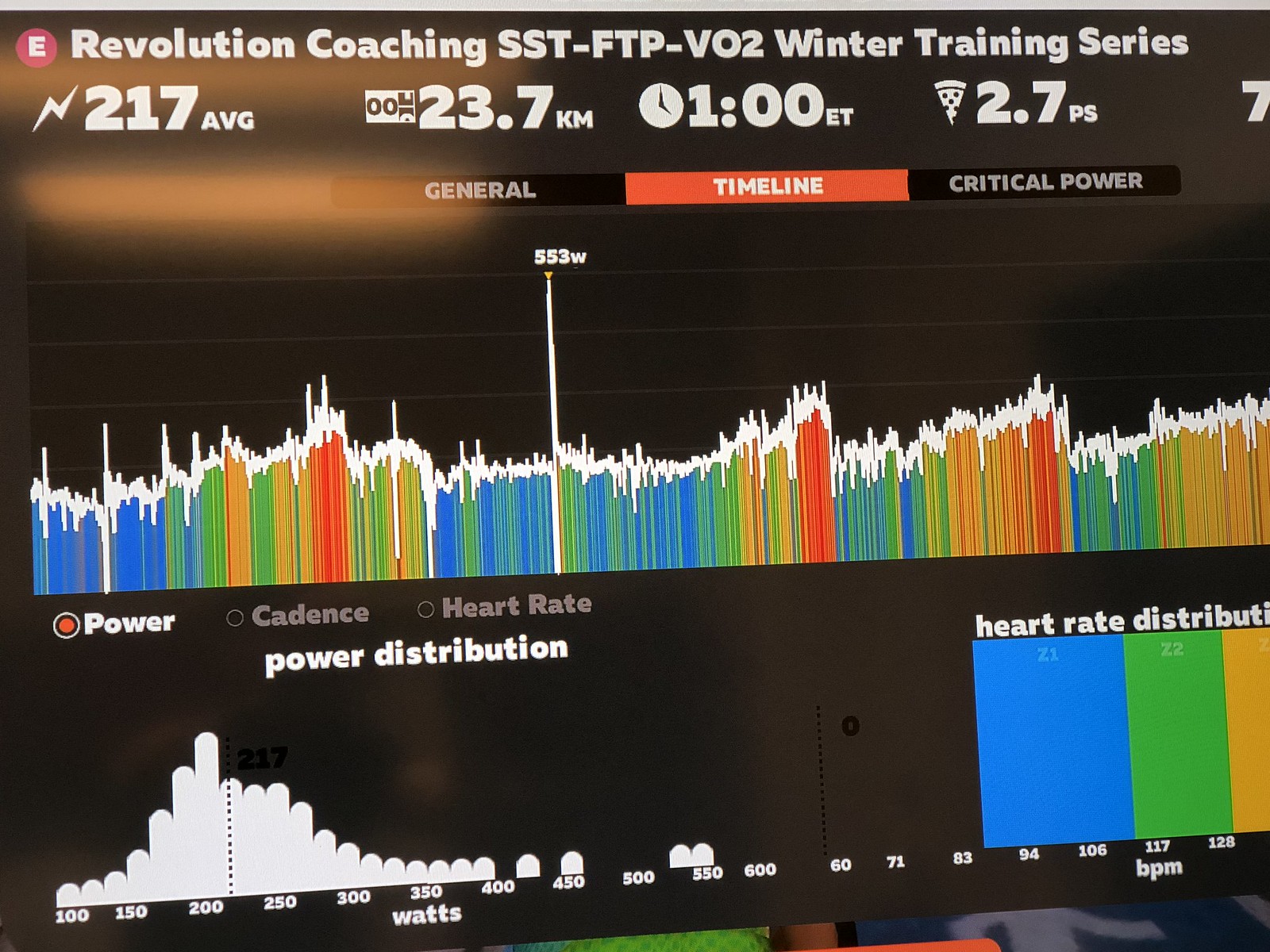The image is a screenshot of a digital dashboard from a workout app with a black background and white text. At the top, in white, it reads "Revolution Coaching SST-FTP-VO2 Winter Training Series." Below this title, the metrics 217 AVG, 23.7 KM, 1:00 ET, and 2.7 PS are displayed. The central section of the dashboard features a graphical timeline with colored lines (blue, orange, yellow) charting various performance metrics, including power, cadence, and heart rate. The tallest line peaks at 553 W. 

At the bottom, there are two main graphs: one showing power distribution, ranging from 100 to 600 watts, with a mean line at 217 watts, and another displaying heart rate distribution, ranging from 60 to 128 BPM, with colors blue, green, and yellow indicating different heart rate zones. Additional labels on the left side of the graph include "power," "cadence," and "heart rate," detailing the measured parameters. Colors used throughout the dashboard include black, white, gray, red, orange, yellow, blue, and green.